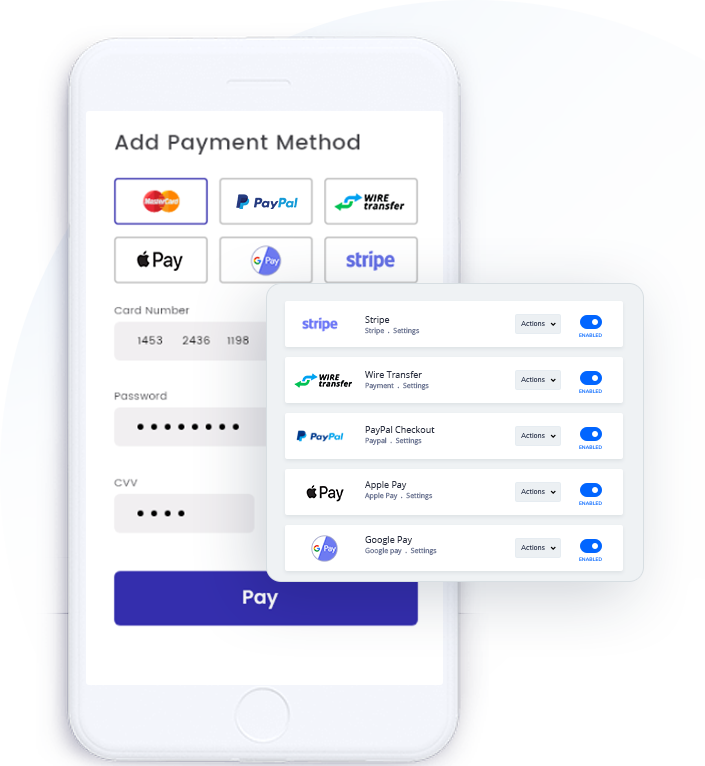The image displays an interface mock-up of a payment method selection screen, occupying the left portion of the image, extending a bit less than two-thirds across. The outline of the interface resembles a phone, glowing softly with subtle gray shadows on each side. To the left, there's a minor circle protruding and disappearing seamlessly, while at the top-right, another circle, in a lighter blue hue, reaches almost to the top and extends horizontally to the right. 

In the center of the phone, originating from the upper and left edges, a small square overlaps halfway, dividing its presence between the phone and the external background on the right. This phone interface features a light blue header, while the main section, starting an inch from the top and extending to an inch from the bottom, is white. 

At the top of this section, in bold black text, the title "Add Payment Method" is displayed. Below this heading, there are six squares arranged in two rows of three, each sporting a blue outline and a white fill. The first row comprises MasterCard on the left, PayPal in the middle, and Wire Transfer on the right. The second row consists of Apple Pay, Google Pay, and Stripe, respectively.

Further down, the form fields begin with "Card Number" in black text, accompanied by a rectangular input box containing a bank number. This is followed by the field labeled "Password" with a gray rectangle displaying password dots. Below it is the "CVV" label and its corresponding rectangular input with four black dots, indicative of security code entry. Finally, at the bottom, a prominent blue button spans from left to right, emblazoned with the word "Pay."

Overlapping this main interface to the left edge of the phone’s frame is a thin-bordered blue tab. This tab contains five horizontally aligned rectangles, separated by slim blue dividers. The top rectangle is marked "Stripe," with settings options to its right, followed by the remaining rectangles for "Wire Transfer," "PayPal," "Apple Pay," and "Google Pay" in descending order. To the right side of this tab, there is a gray button labeled "Actions" in black, and below it, a small blue circle with a white dot, denoting "Disabled" status.